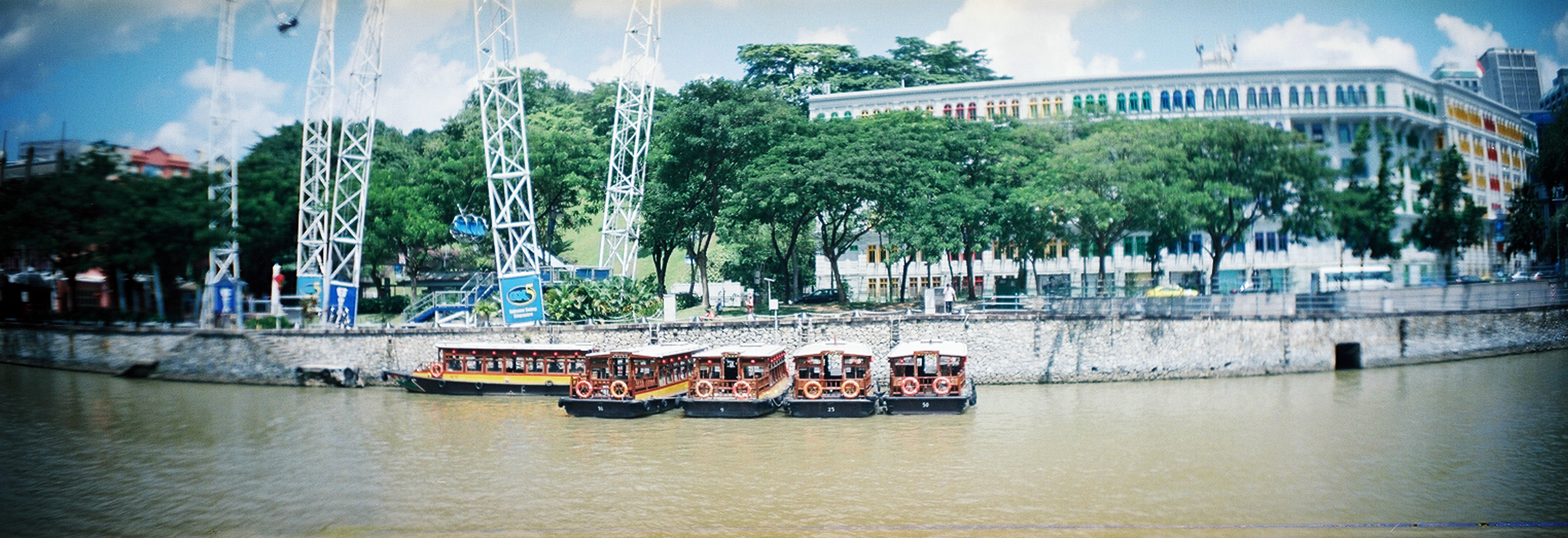The photograph captures a vibrant, bustling riverside scene saturated with detail. From left to right, the foreground reveals a muddy, light-brown river where five passenger ferry boats, identical in design, are aligned. These flat-bottom boats feature a distinctive color scheme: black hulls transitioning to vibrant yellow midsections, capped with light gray canopies supported by red bars. Notably, one of the boats is oriented sideways as if navigating out of the line.

The riverbank is fortified by a substantial concrete wall that displays shades of tan and gray. Behind this barrier, a lush tree line with varying shades of green foliage stretches along the scene, enhancing the natural beauty of the setting. Prominently, white cranes with blue signs affixed to their bases rise into an azure sky peppered with white clouds, signaling industrial activity nearby.

In the background, a five-story building adorned with an array of colorful banners—blue, green, red, yellow, and orange—adds a splash of vibrancy to the urban landscape. Its uppermost rows of arched windows, in hues of blue and light blue, overlook the river. Further in the distance, a cityscape with towering skyscrapers punctuates the horizon, completing the picturesque yet industrious scene. The presence of life preservers affixed to the boats hints at the readiness for safe passenger transport, making the photograph an intricate tapestry of natural beauty, human ingenuity, and urban development.